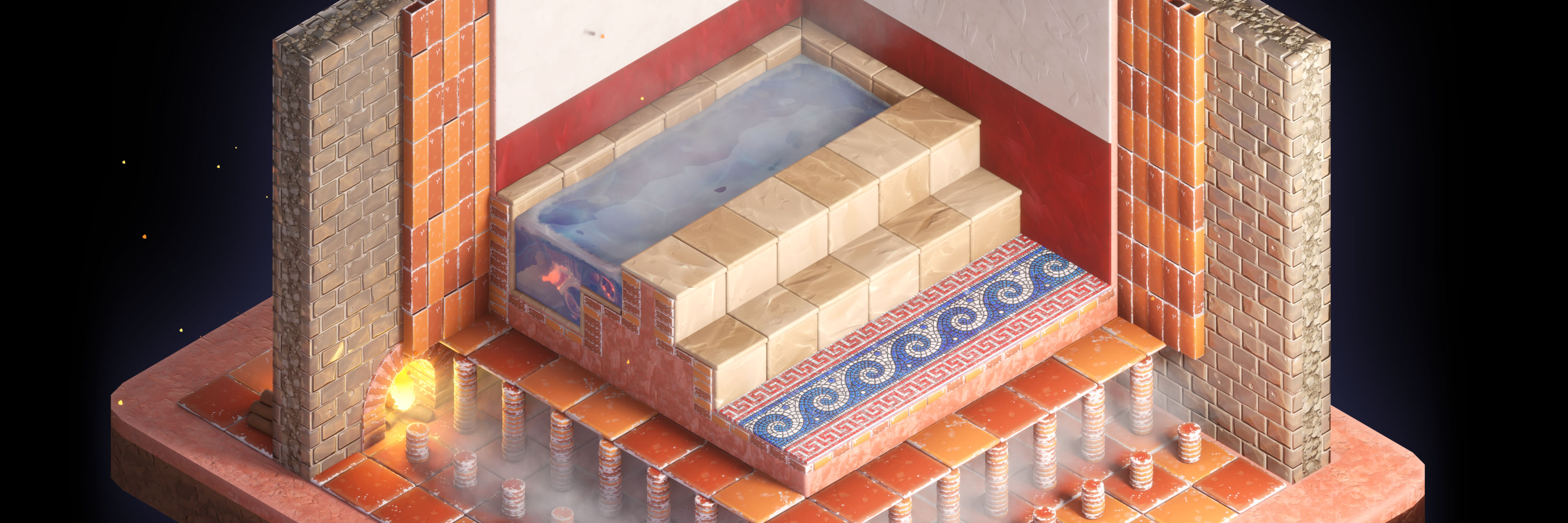The image presents a detailed three-dimensional model showcasing a small architectural structure. The predominant color theme is shades of red and orange, which adorn various elements of the model. The model appears to depict a hot tub or small pool, built on a multi-layered platform. The base layer is made of block stone or tile, elevated by pillars that are distinctly orange. Another layer features a wave pattern, suggesting ocean waves, crafted meticulously with small tiles. Above this, the final platform supports the hot tub or pool, filled with a small amount of water.

The structure is set against a stark, solid black background, which accentuates its vibrant colors. Notable details include brick walls with red and orange tiles, transitioning to a white section, and marbled steps patterned with waves leading up to the tub area. The left side of the image features what seems to be a light source, possibly a furnace or chimney, adding a glow that highlights the base of the model. This meticulous depiction likely serves as a small-scale representation or display model, illustrating the final design of the intended structure.